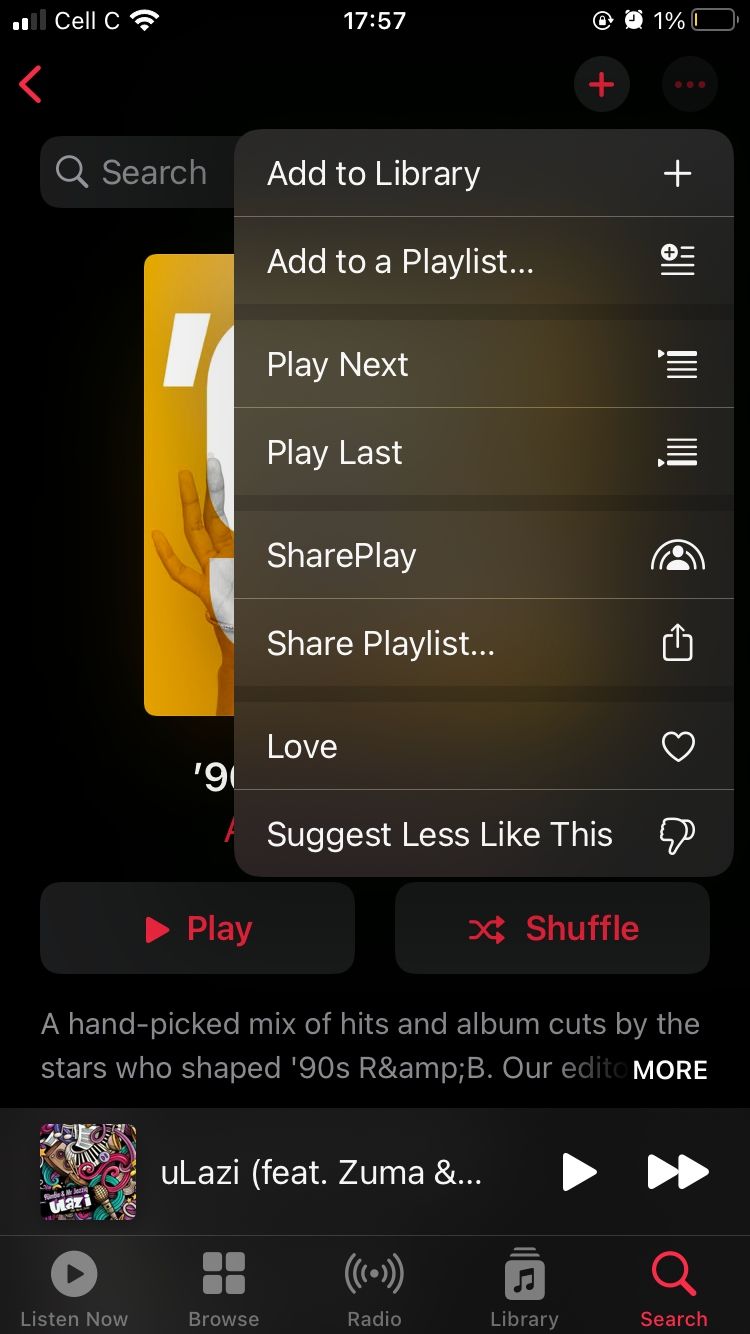**Detailed Caption:**

The screenshot appears to be from a mobile device, likely showcasing a musical application, as indicated by various elements on the screen. The background is predominantly black, enhancing the contrast of the interface elements.

In the upper left-hand corner, the phone’s status indicators are displayed, starting with a cell signal showing two out of four white bars labeled "Cell C." Next to it, the Wi-Fi signal strength is shown. The current time is centrally displayed as "17:57." Moving to the upper right-hand corner, several icons are visible: a screen rotation lock icon, an alarm clock icon, and a nearly depleted battery icon showing just 1% charge with a thin white sliver of remaining energy.

Below these status icons, a red arrow pointing to the left appears, symbolizing a back function. On the far right, we see a red plus symbol and a red icon with three horizontal dots, typically indicating additional options or a menu.

The search bar, which is black with a gray magnifying glass icon and the word "Search," is currently overlaid by a sub-menu. The menu options are displayed in white text and include: Text, Add to Library, Add to Playlist, Play Next, Play Last, Share Play, Share Playlist, Love, and Suggest Less Like This.

In the background of the menu, the image of an album cover is partially visible. Its main color appears to be yellow, and it includes a comma, possibly the number nine, and a right hand in an open position. Below the album art, the number "90" is visible, indicating perhaps the theme or era of the music.

Further down, two black buttons with red text are present. The first button on the left says "Play," and the second button says "Shuffle." Just below this, a caption reads: "A hand-picked mix of hits and albums cut by the stars who shaped the 90s are," but the text is partially cut off.

Further details reveal information about the currently playing song. A small thumbnail image of an album is displayed next to the text "Ulazi," followed by "featuring Zuma" (again, part of the text is cut off). Below this, a Play button and a Fast Forward button are visible.

At the bottom row of the interface, a navigation menu is present with five icons. From left to right: "Listen Now," "Browse," "Radio," "Library," and a highlighted red "Search" icon. The first four icons are in gray, indicating they are not currently selected.